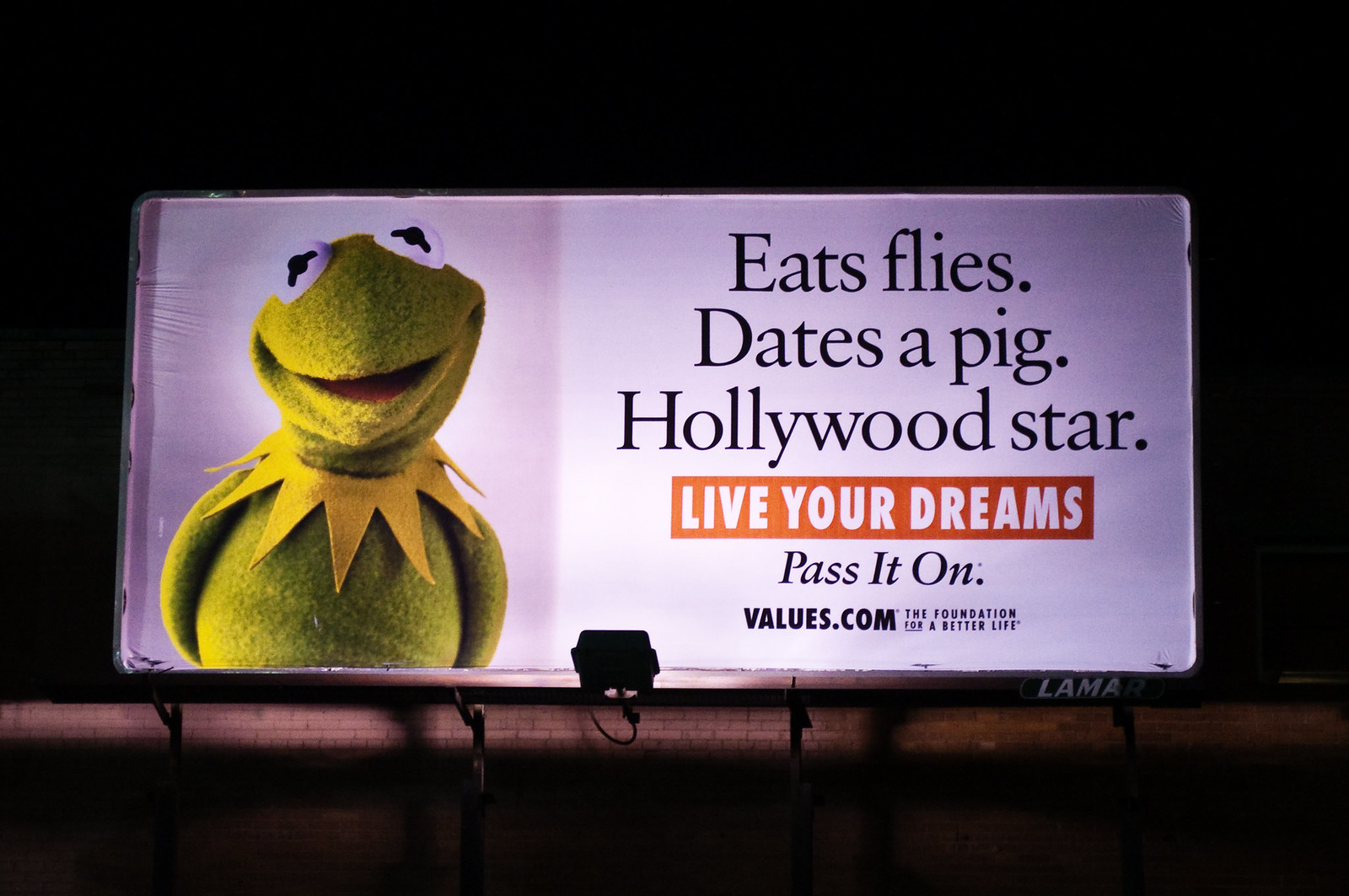This nighttime photograph features a billboard illuminated by a bright spotlight positioned below it. The billboard prominently displays an image of Kermit the Frog on the left side. The right side of the billboard contains text in black that reads, "Eats flies. Dates a pig. Hollywood star." The background of the billboard is white. Below the text is a small red box with the encouraging message, "Live your dreams." Beneath this, in smaller black text, it reads, "Pass it on. Values.com. The foundation for a better life." At the very bottom of the billboard, the word "Llama" is visible in white letters. The billboard appears to be mounted against a brick wall.